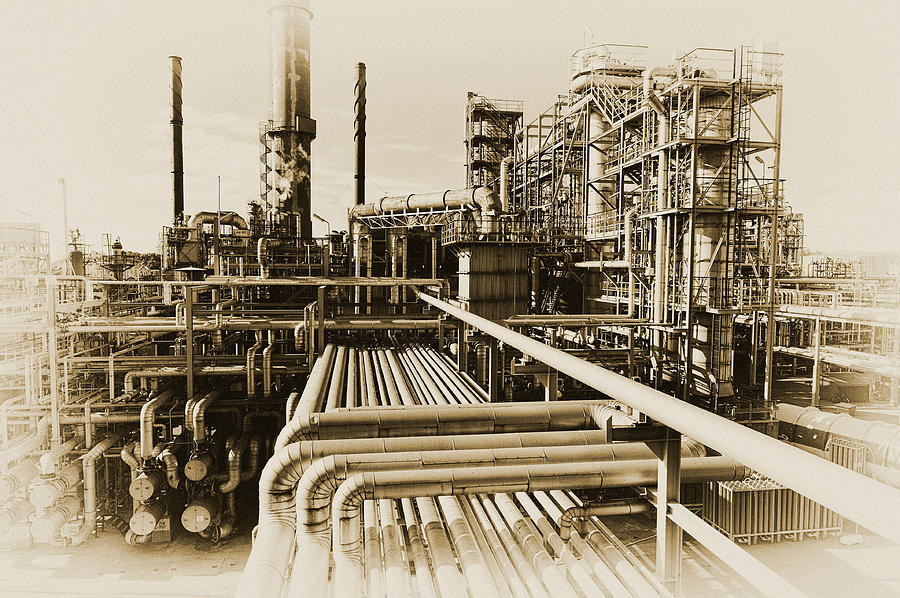The image is a black-and-white, sepia-toned photograph of a large industrial factory, reminiscent of the "Rust" map from the 2009 video game Call of Duty: Modern Warfare 2. In the foreground, several large pipe structures crisscross, extending vertically and horizontally, leading towards the factory. The factory itself is enveloped in a maze of metallic scaffolding, stairways, and bridges, giving it a complex and robust industrial appearance. Prominent in the scene are multiple large pipes and smokestacks protruding from the main structure, emphasizing its function of possibly handling gas, water treatment, or electrical processes. The overall composition of pipes varies in size, with some extending high into the air, creating a dense network of metal surfaces and intricate designs that dominate the scene.